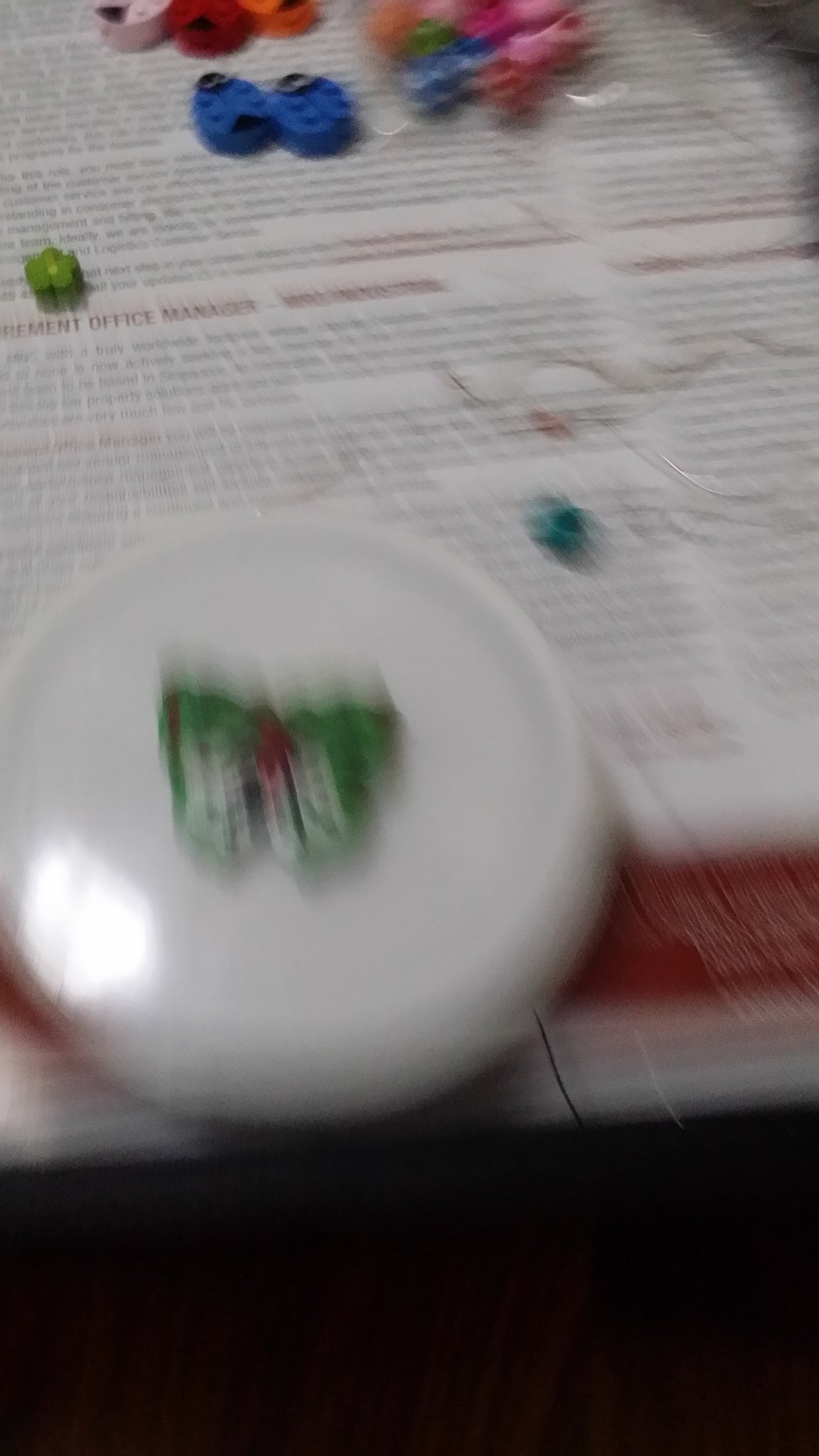In this blurred photograph, a cluttered surface is depicted with various items atop what seems to be a magazine or newspaper. Dominating the center, there is a plate featuring a butterfly with green wings and a red center. Surrounding the plate are numerous small, round objects in an array of colors including green, sky blue, dark blue, red, pink, and orange. These objects appear to have buttons, though their exact nature is indistinguishable due to the blurriness. The only discernible text on the paper is "office manager." The image is significantly out of focus, suggesting the camera was moved while the picture was taken, making it difficult to ascertain additional details or the floor surface.